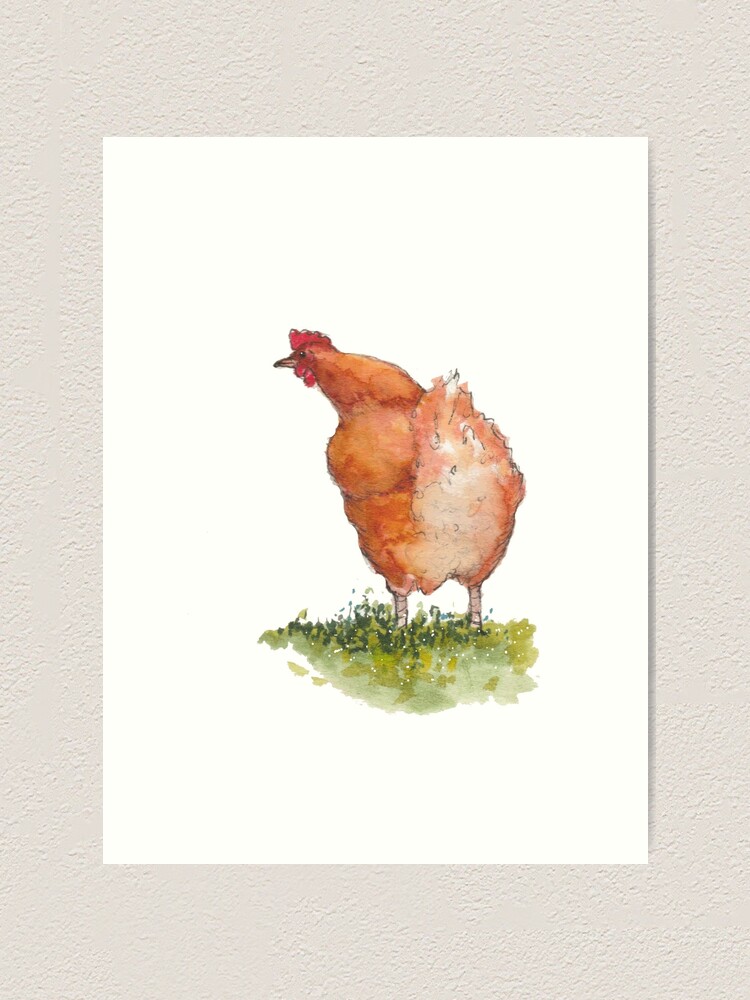The image is a vertical rectangular drawing of a rooster, presented on a white piece of paper against a cream-colored, textured matting, all set against a gray background. The rooster is depicted with our view from behind, showcasing its rear and slightly raised tail feathers. Its body exhibits a spectrum of brown to orangey-red hues, transitioning to white on the feathers under its tail. The head is turned to the left, featuring a prominent red comb on top and a red wattle beneath its beak. The beak itself is brown. At the bottom of the image, the rooster's feet are partially obscured by loosely sketched green grass, adding a touch of natural detail to the drawing.